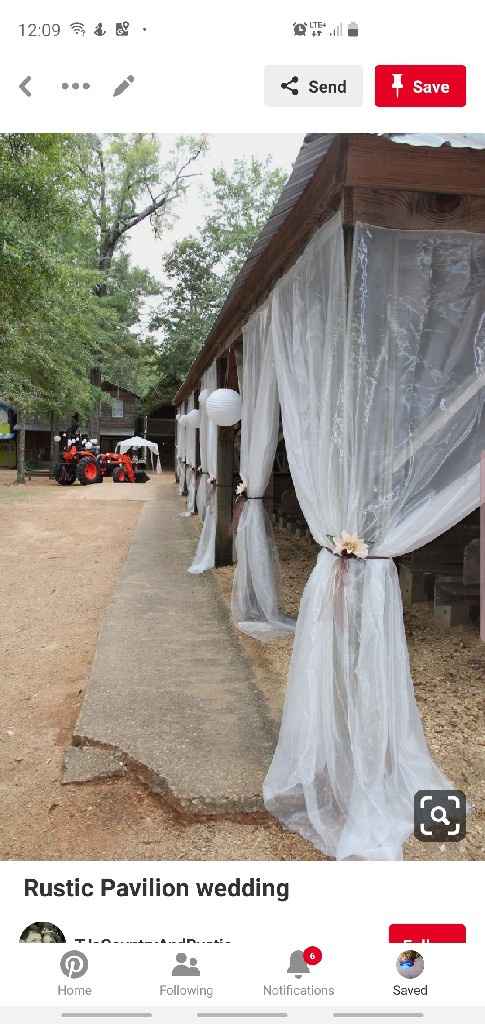This image is a detailed screenshot from a mobile phone displaying a photo on Pinterest. The photo showcases a wedding setup under a rustic pavilion in an outdoor field with a dirt floor and surrounded by trees. The pavilion, made of dark wood, features white tulle draped from its roof and tied around each post with bouquets of white flowers. White balloons add to the festive decor. In the background, an orange tractor and a small white tent are visible, presumably part of the wedding setting. The text below the image reads "Rustic Pavilion Wedding," indicating this as an inspiring wedding venue idea. The phone's interface shows time, notifications, battery life, and Pinterest buttons for sending, saving the image, and navigation tabs like home, following, notifications, and saved.